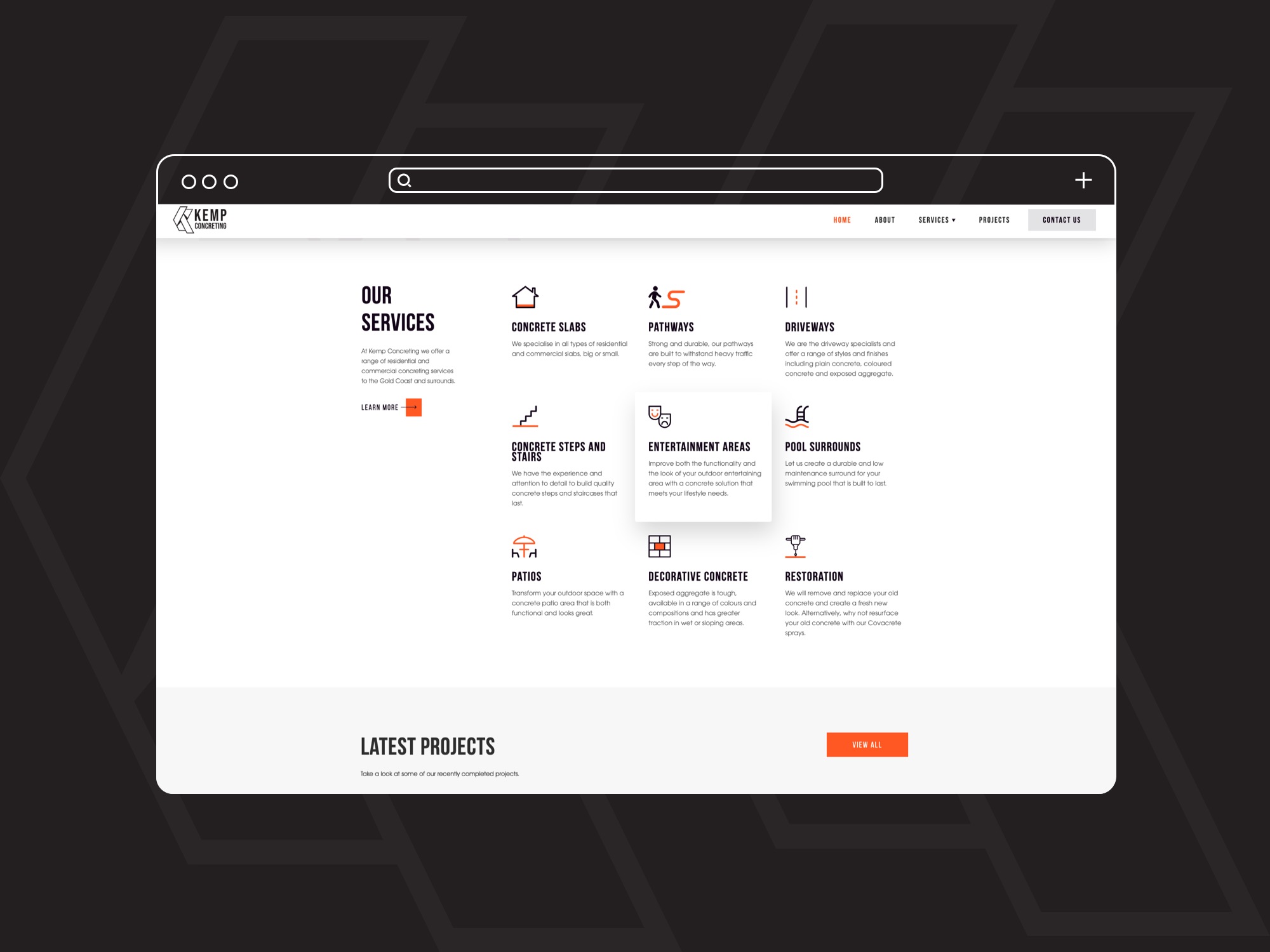The image presents a screenshot displayed on a rectangular black background. Centrally positioned is a white screenshot bordered by a black header. On the upper left of this header, there are three white outlined circles. At the center, a search bar featuring a white magnifying glass icon is visible, and in the upper right corner, a plus sign is evident. Directly below the header, a white banner showcases the website name "Kemp Concreting" in black text, accompanied by a geometric-style logo on the left. To the right of this banner, a horizontal menu is displayed, with buttons labeled: "Home" in red, "About," "Services" (which includes a pull-down arrow), "Projects," and a highlighted "Contact Us."

Below the menu, bold black text reads "Our Services," followed by specific service offerings listed from left to right: "Concrete Slabs," "Pathways," and "Driveways." On the subsequent line, additional services include "Concrete Stairs," "Entertainment Areas," and "Pool Surrounds," all presented in bold black text.